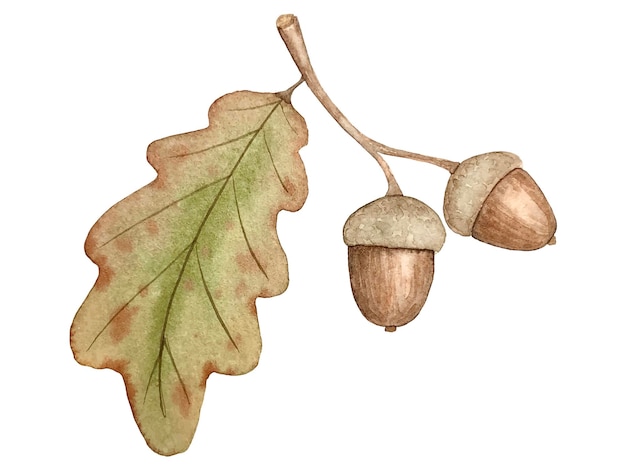This image resembles clip art frequently used in presentations or digital content. It features a detailed drawing of an oak branch with a faded green leaf and a smaller attached branch bearing two uniformly-sized acorns. The brown hue of the acorns matches the color of the branch. Upon close examination, the illustration captures the nuanced beauty of a common sight in nature and evokes thoughts of a squirrel’s cherished treat. The leaf appears to be slowly withering, adding a touch of realism and poignant beauty to the depiction.